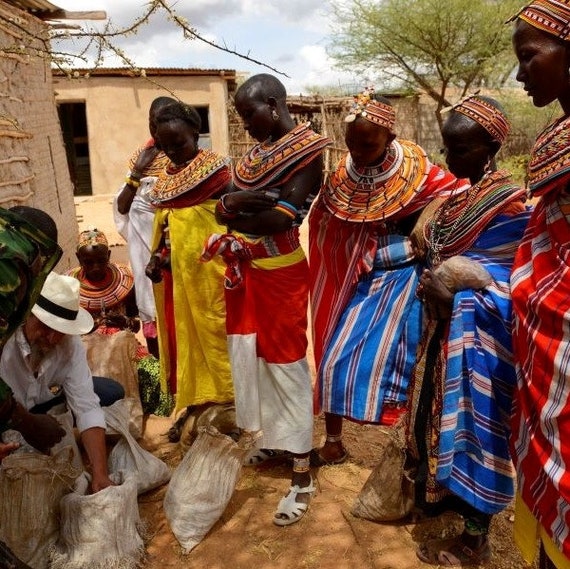The square photograph captures a vivid scene in an African setting, indicated by the traditional garb of the seven individuals present, comprising both men and women. They are adorned in colorful, robe-like attire, featuring hues of blue, red, yellow, and white, with intricate pinstripes. Each person wears an elaborate, woven decorative piece around their neck, extending over their shoulders, and some complement their outfits with matching headbands and earrings. They stand on a clay-like surface with brick-like structures with flat roofs and an acacia tree in the background, adding a distinct regional touch.

Central to the image, a Caucasian man, possibly American or European, dressed in a broad-rimmed white hat with a black band and a white long-sleeved shirt rolled up to his elbows, draws the group's attention. Leaning slightly, he reaches into an open burlap sack and white cloth bag, suggesting he is demonstrating or presenting something to the onlookers. The scene exudes a sense of interaction and exchange, grounded in a culturally rich environment.